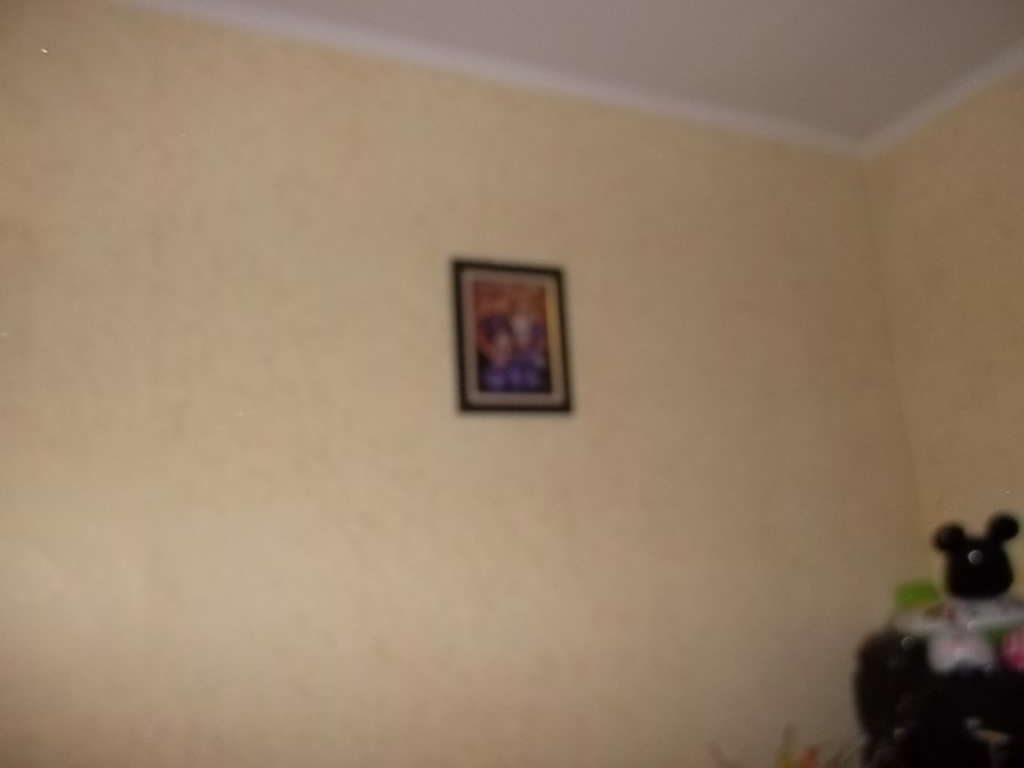This photograph captures an indoor scene in a house, notable for its distinct 80s or 90s aesthetic and characteristic blurriness. The image focuses on two walls and a section of the ceiling where the walls converge. The ceiling is a clean white, while the walls exhibit a yellowish-cream tone. The main wall, occupying most of the photograph, features a black-framed picture, although the exact details of the image within the frame are obscured and appear to depict two people. In the corner to the right, there's a small part of an adjoining wall. On a table positioned in this corner, a black ceramic bunny figurine is faintly visible. The overall setting exudes a nostalgic feel, heightened by the photograph’s lack of clarity.